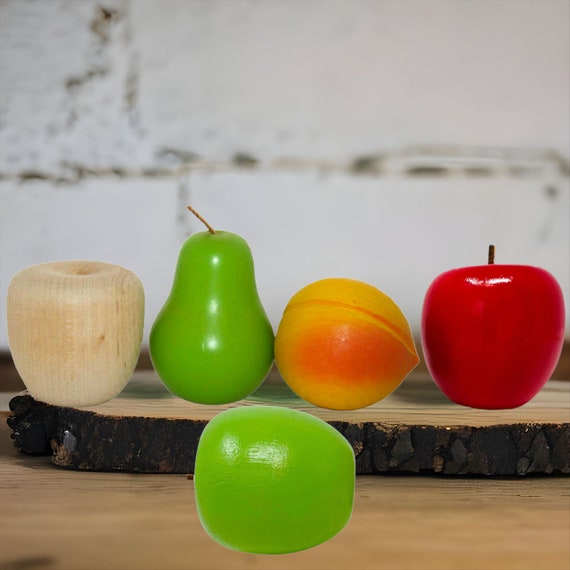The photograph showcases an arrangement of various styles of artificial fruit displayed in front of a blurred, vintage white brick wall. In the foreground, a shiny green apple with a tiny brown stem, angled to the left, lies on its side on a plank of wood. Behind this, a rustic wooden bark round cutout serves as a platform for four other pieces of fake fruit. Starting from the left, there is an unpainted wooden apple, followed by a shiny green pear with a stem pointing left. Next to the pear is a yellow and orange apricot lying on its side, and finally, a shiny red apple with a small brown stem sits upright. Each piece of fruit is meticulously detailed and polished, contributing to the overall aesthetic of the display.